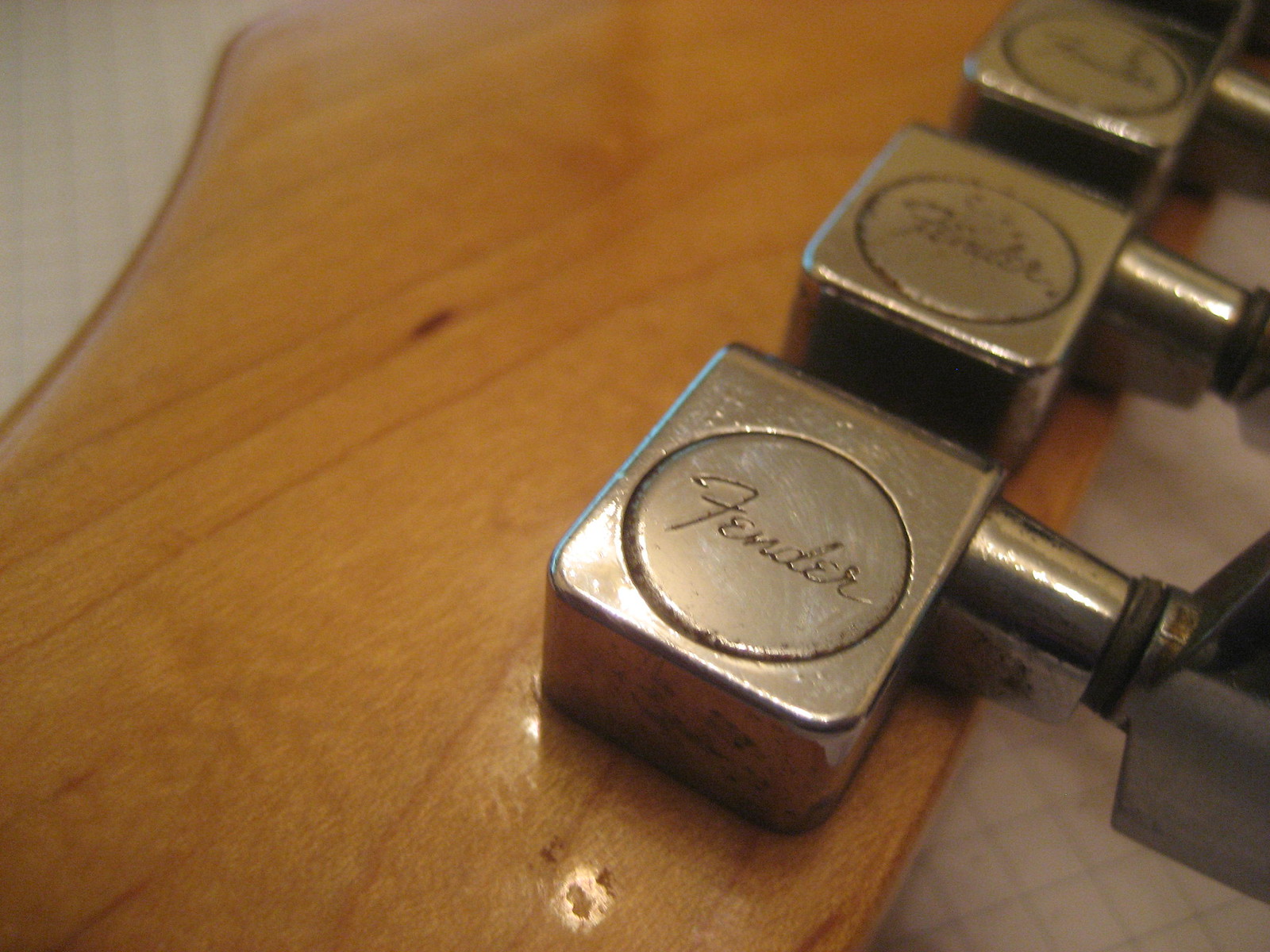The close-up image captures a reflective silver metal tuning mechanism stamped with the word "FENDER" encircled by a ring, indicative of the well-known guitar brand. This metal device, likely part of a guitar or similar string instrument, is positioned on a light brown wooden surface with intricate grain textures, partially extending beyond the edge to the right. The guitar's tuning keys are visible to the right, leading into a box that features the Fender branding. The photograph is taken indoors, with a subtle yellowish hue illuminating the scene and casting reflections on the polished metal. The backdrop showcases a white wall, enhancing the instrument’s craftsmanship and the warm tones of the wood.